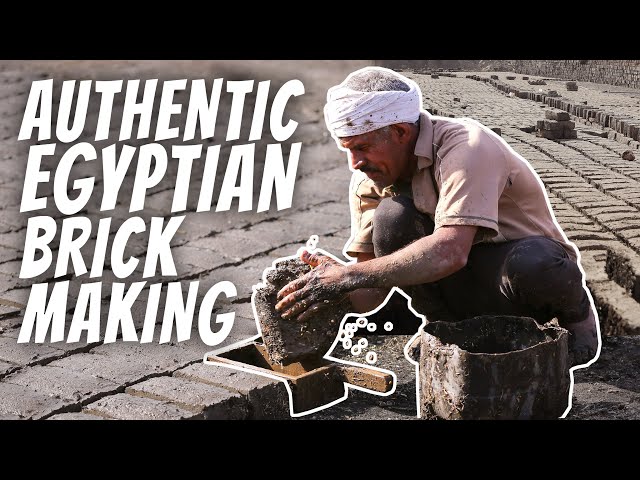The image depicts an older man with white hair engaged in the traditional craft of brick making in an expansive field dotted with bricks. He is kneeling down, focused on his work, wearing a tan-colored polo shirt and black pants, with a white bandana wrapped around his head. His hands are visibly muddy as he handles a brick-making mold designed for shaping the bricks. Next to him lies a weathered, beaten silver bucket likely used for mixing cement. The man is surrounded by rows upon rows of gray bricks that stretch into the background. The setting is framed with thicker black lines at the top and bottom of the image. In white capital letters on the left side, the caption reads: "AUTHENTIC EGYPTIAN BRICKMAKING."